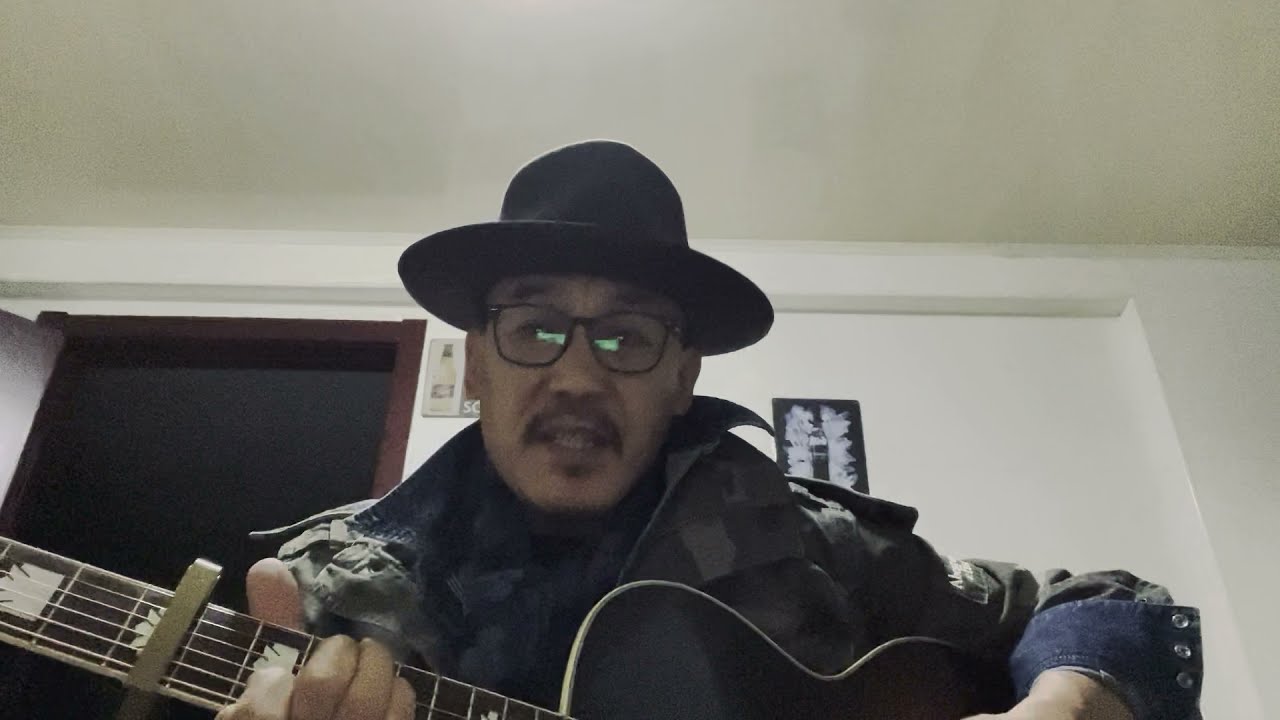In the image, a man focuses intently as he looks down at his computer screen while playing a black guitar with white trim. He is dressed in a camouflage-colored jacket with distinctive blue wrist cuffs, and he wears a black fedora and black-rimmed glasses that reflect the computer monitor. The man's facial features are highlighted by his black mustache and a small patch of hair on his chin. An open doorway with a dark brown wood frame is visible behind him, leading into a shadowy, indistinct room. The wall and ceiling are both white, and there is a piece of artwork bordered in black with white smudges hanging on the wall. The composition gives a close-up view of the upper portion of his body and the top part of the guitar, emphasizing his concentrated expression and the reflective quality of his glasses.